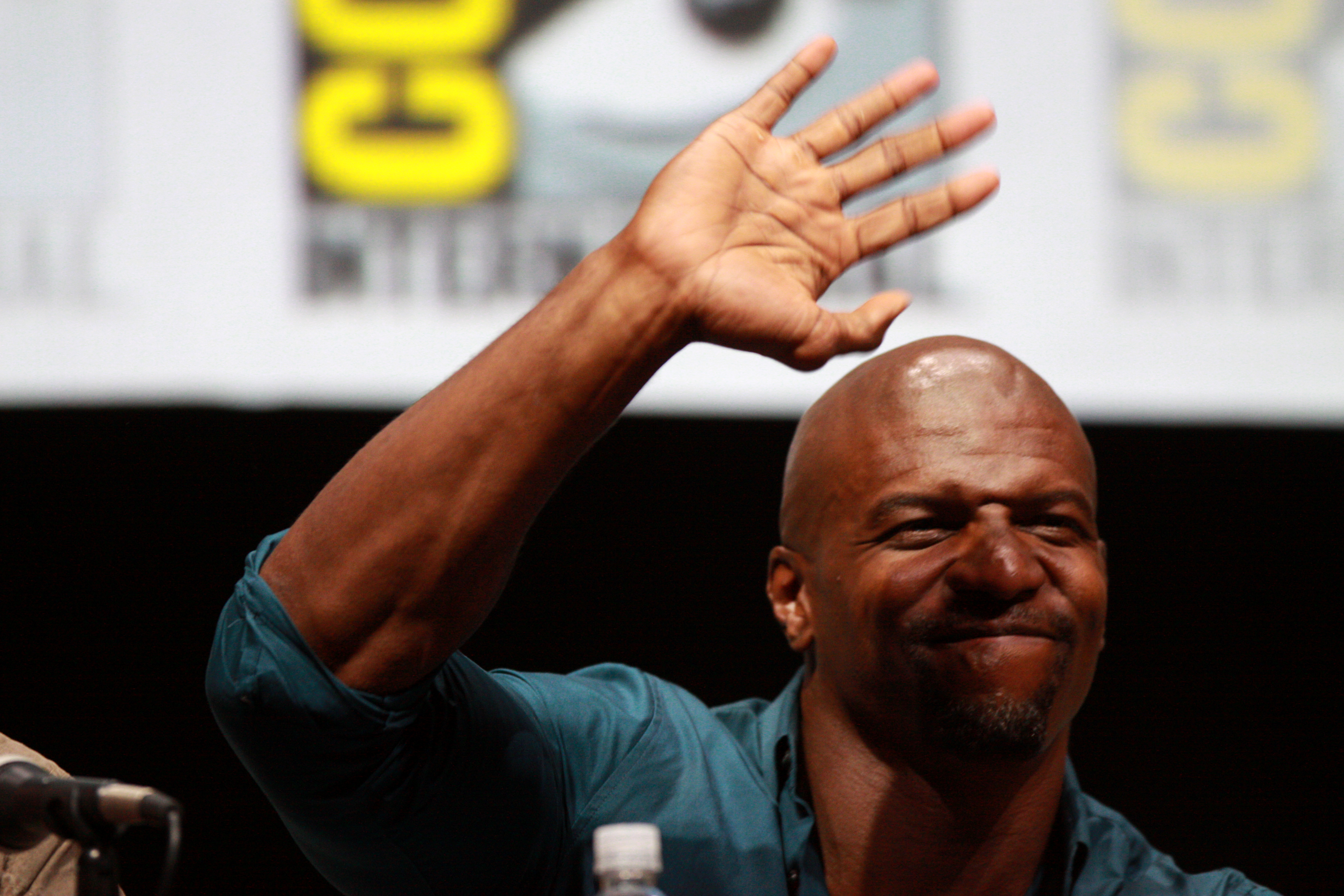The photograph depicts Terry Crews, a black male actor, at a comic-con convention. He is seated on a stage panel and is dressed in a dark teal, collared shirt with sleeves rolled up to his elbows, accentuating the muscles in his forearm. He is waving with his right hand raised above his head, palm facing outwards, casting a shadow on his smiling face. His head is shaved bald, and he sports a neatly trimmed black goatee. Terry is looking slightly to the right, squinting his eyes a bit as he smiles. The background features a partially visible San Diego Comic Con banner, with the recognizable yellow "C" from the logo, set against a predominantly black lower half. To the left of the image, a microphone stands on a higher surface, and a cropped-out person in a tan shirt is partially visible. A plastic bottle's cap is seen at the center bottom of the image, contributing to the setting's casual yet organized atmosphere.